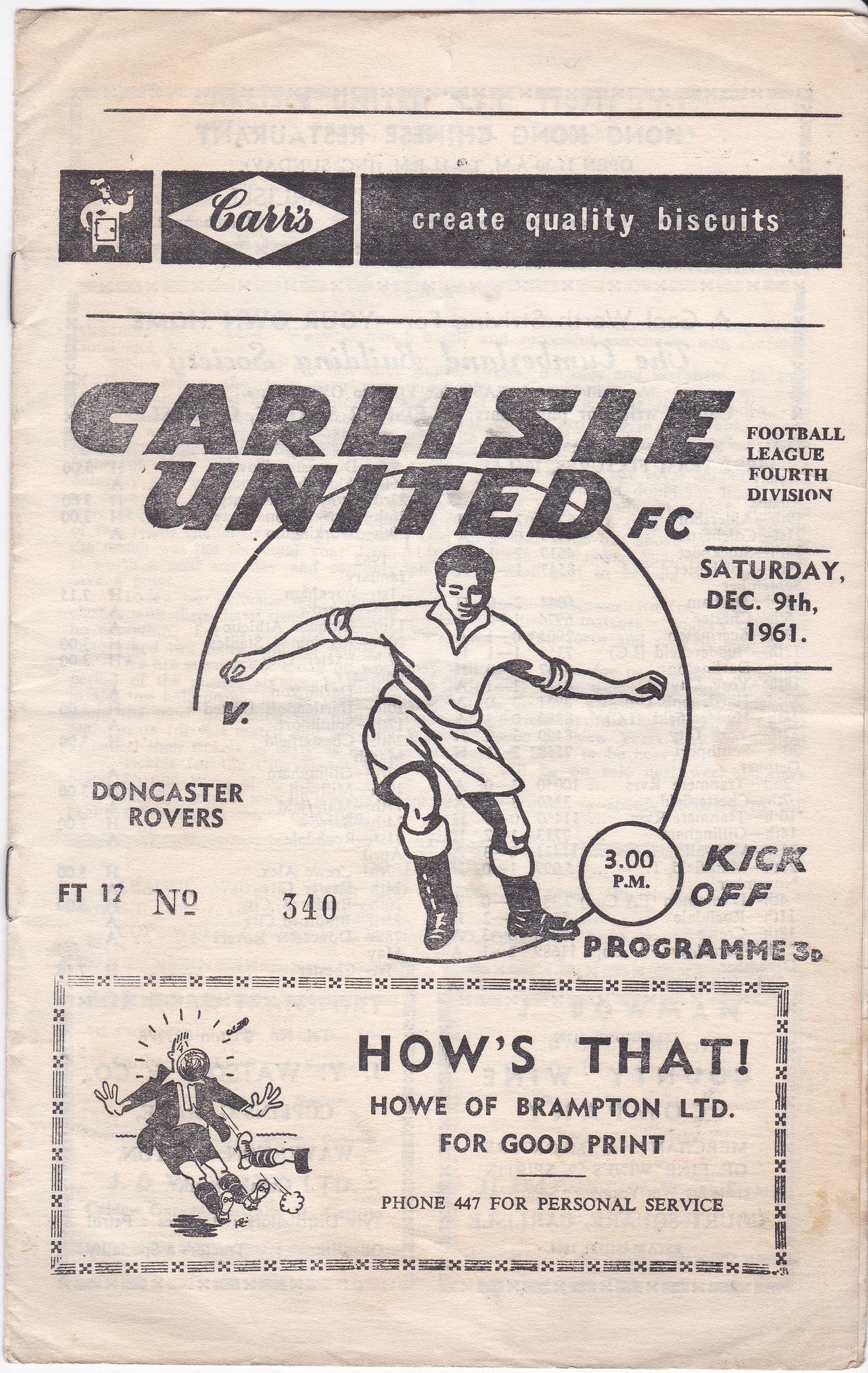The image is a black-and-white cover of an old sports program, specifically for a football (soccer) match held on Saturday, December 9, 1961. The program cover, which is slightly tattered and creased, is held together by two staples on the left side. 

At the top of the cover, there is an advertisement that reads "CARRS create quality biscuits." Below this, prominently displayed, is a header that says "Carlisle United FC vs Doncaster Rovers," indicating a match happening at 3 p.m. The cost of the program is noted as 3 pence.

The main illustration features a drawing of a young boy in a soccer costume, encapsulated in a circle. At the bottom, there is another advertisement within a rectangle, depicting a person falling down and bearing the text: "How's that? How, H-O-W-E, of Brampton Limited, for good print. Phone 447 for personal service." 

Additional text includes "Football League 4th Division," aligning with the era and nature of the program.